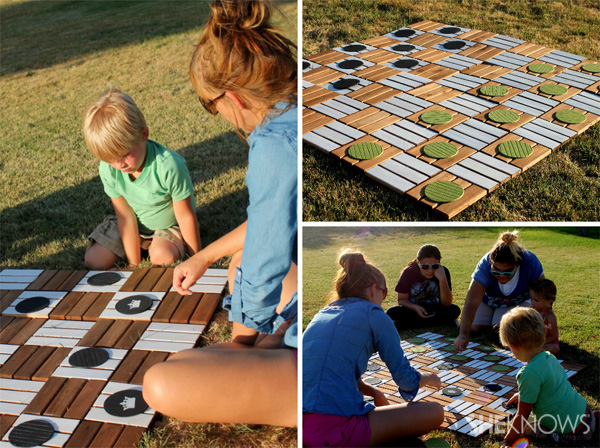The composite image merges three photographs depicting a family engaged in a lively outdoor game of oversized wooden checkers on a grassy lawn. The left-hand photograph features a red-haired woman in a long-sleeve, jean-colored shirt and shorts, sitting to the far right. In the center, a young blonde boy wearing a mint green T-shirt and cargo shorts is deeply engrossed in the game. The checkerboard consists of alternating three-paneled brown and white wooden squares with large green and black pieces, some of which are crowned with white symbols indicating kings.

The top-right photograph highlights the checkerboard itself, resting on the grass, showing black pieces on the left side and pea-green pieces on the right. Finally, the bottom-right photograph reveals five people gathered around the game. A woman with a blue shirt and pink shorts, her hair in a bun, and a young blonde boy in a mint green T-shirt both have their backs to the viewer. Three individuals, facing the viewer from across the board, include an adolescent girl with a ponytail and sunglasses in a maroon shirt, an older blonde woman with blue glasses in a blue T-shirt, and another young girl, partially obscured by the boy.

The entire scene exudes a sense of family fun and togetherness, set against the backdrop of a sunlit day, with the words "She Knows" subtly overlaid at the bottom in white, translucent text.